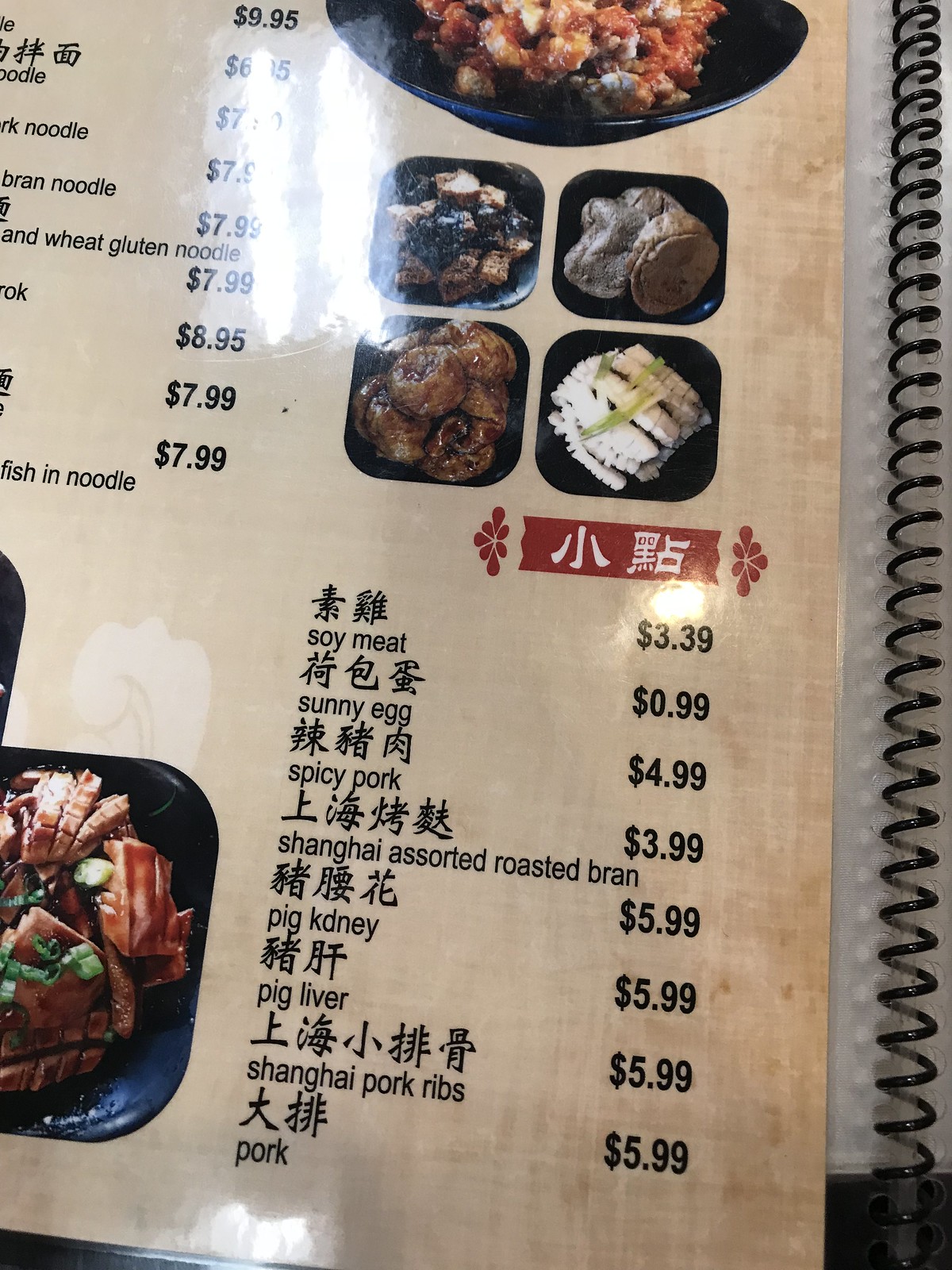The image captures a detailed view of a Chinese restaurant menu, which is laminated and set against a beige background. At the top of the menu, there is a colorful photograph of a meat dish served in a black bowl, tantalizing and appetizing in appearance. Directly below this centerpiece image are four smaller squares, each showcasing different ingredients, rice, and a variety of meats, offering a visual introduction to some of the dishes available.

Down both sides of the menu is an extensive list of food items, carefully organized with Chinese characters written above each English translation, followed by the respective prices to the right. Although the top of the menu is slightly cut off, the bottom portion provides a clear list of items, including:
- Soy Meat: $3.39
- Sunny Egg: $0.99
- Spicy Pork: $4.99
- Shanghai Assorted Roasted Bran: $3.99
- Pig Kidney: $5.99
- Pig Liver: $5.99
- Shanghai Pork Ribs: $5.99
- Pork: $5.99

Centrally positioned on the menu is a striking red banner adorned with floral designs on either side. In the middle of this banner, white Chinese lettering adds a traditional touch, emphasizing the cultural authenticity of the restaurant's offerings.